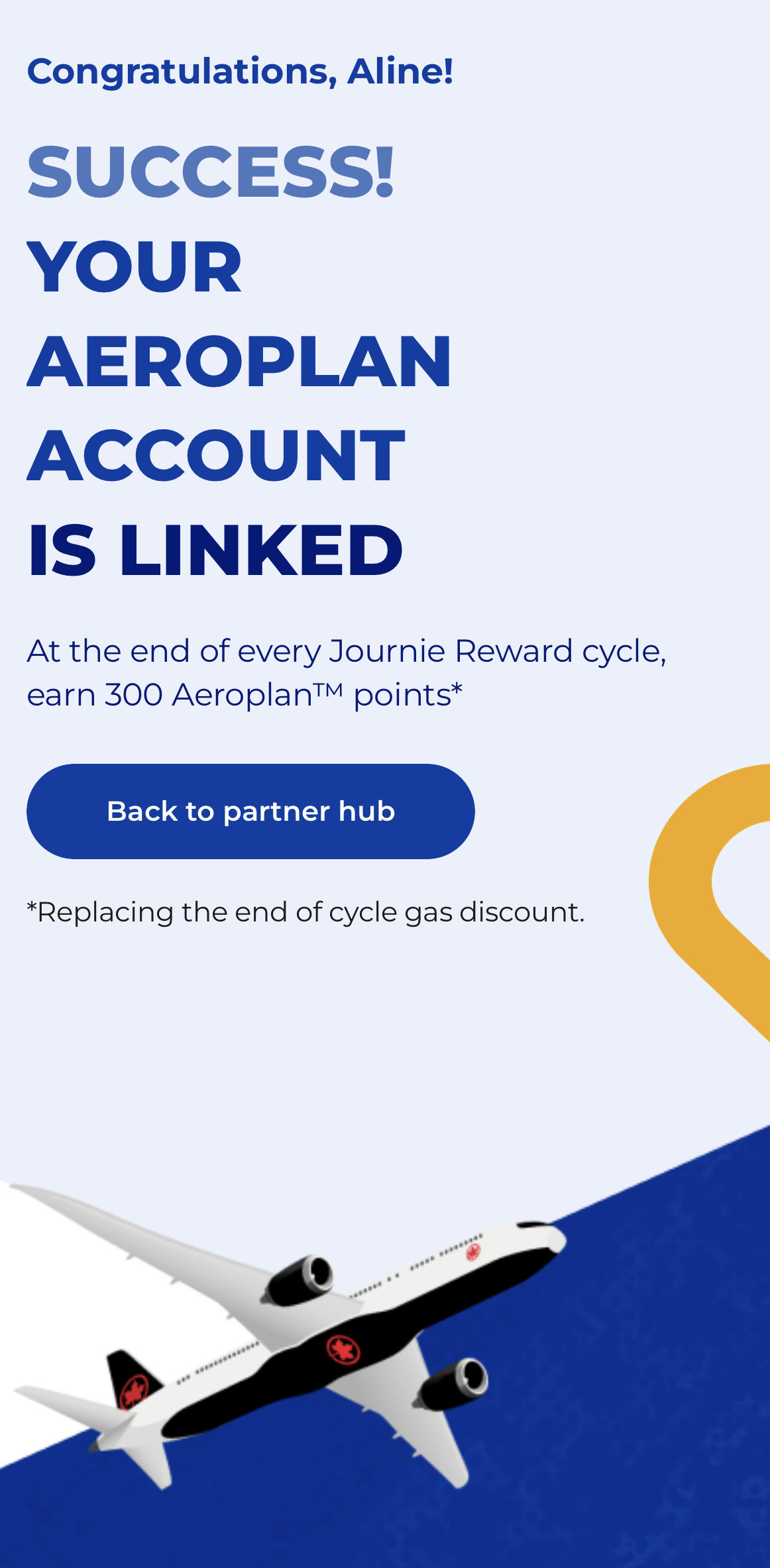The digital image prominently features a congratulatory message with the text: "Congratulations, A-Line, Success. Your AeroPlan account is linked." The message indicates that upon the completion of each journey reward cycle, the user will earn 300 AeroPlan points, noted with an asterisk indicating additional details. The image includes a blue and white button labeled "Back to Partner Hub." Beneath this button, another sentence marked with an asterisk mentions, "replacing the end of cycle gas discount."

The backdrop of the image showcases a large commercial airliner. The aircraft is primarily white with a black underbelly and white wings. Its tail is also white, adorned with a vivid red maple leaf – the emblem of Canada. The sleek and modern design of the plane underscores the airline's commitment to excellence and national pride.